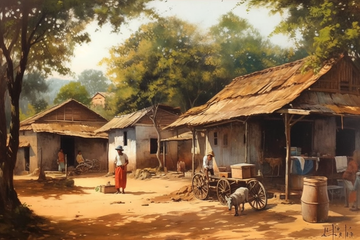This detailed painting depicts a rustic village scene with three older-style houses prominently in view. Two of the houses are white with thatched roofs, while the third is brown. In the center foreground, a person in a white loose-fitting shirt paired with a red skirt stands next to one of the houses, surrounded by various household items such as baskets and buckets filled with clothes scattered on the porch. The ground is predominantly brown and yellow dirt, devoid of grass.

Further adding to the scene's rural charm, a traditional wooden wagon fitted with aged tires sits near the houses, possibly hitched to a small donkey or goat seen close by. A barrel occupies a spot in the front yard, and a person dressed in orange pants and a blue cap can be noticed further back, seemingly engaged in an activity. The backdrop is lush with green trees under a cloudy white and blue sky, portraying an afternoon ambiance. An additional house is faintly visible in the distance, and several people are indistinctly noted around the third house, adding life to this pastoral setting.